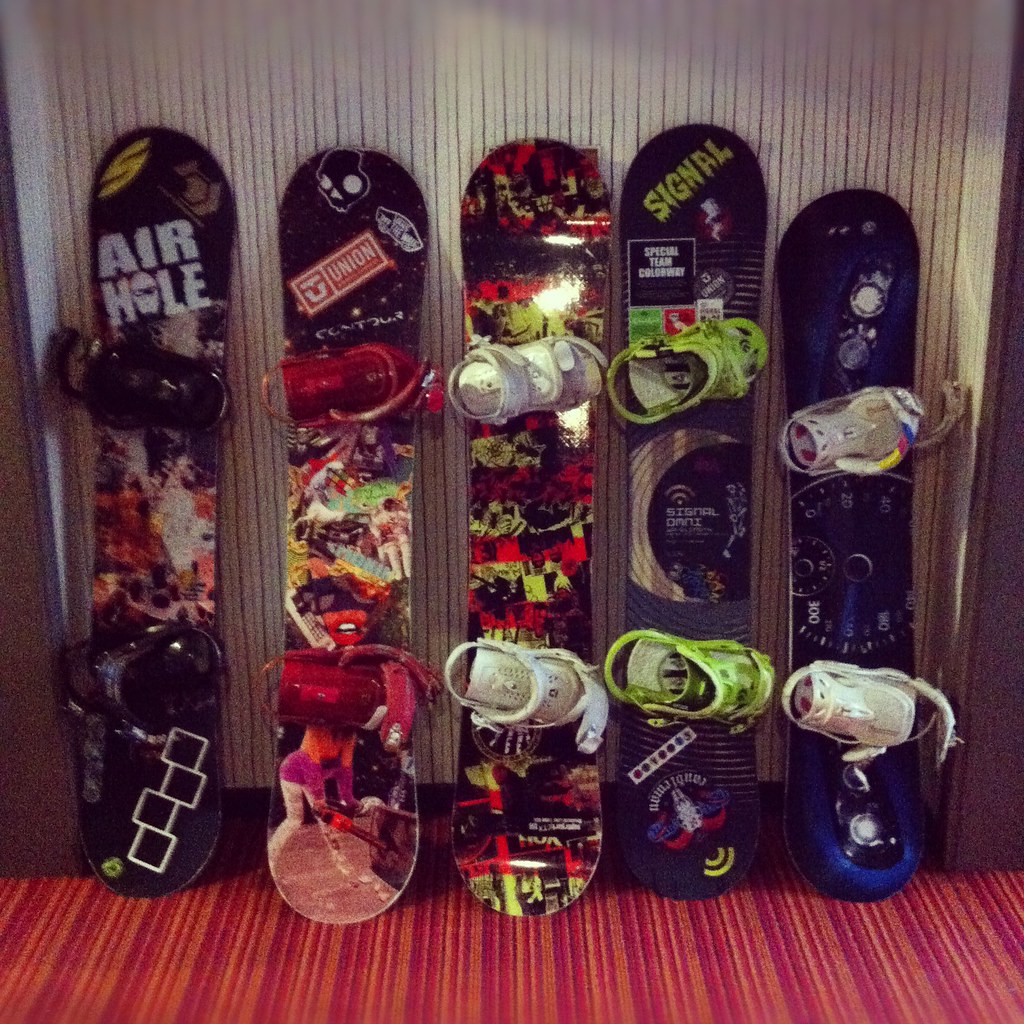This image captures five colorful snowboards standing upright against what appears to be white curtains with thin black stripes. The floor below them is an orange and magenta-colored carpet. Each snowboard has a pair of boots attached, adding to the vibrant array of colors that include green, red, blue, yellow, and lime. From left to right, the first snowboard has "Airhole" printed on it, featuring black bindings. The second snowboard is marked with "Union" in red, accompanied by red bindings. The middle board showcases a combination of black, yellow, and red with white bindings. Next is a board highlighted with "Signal" in lime color, and matching lime bindings. The final snowboard on the right is predominantly royal blue with white bindings.